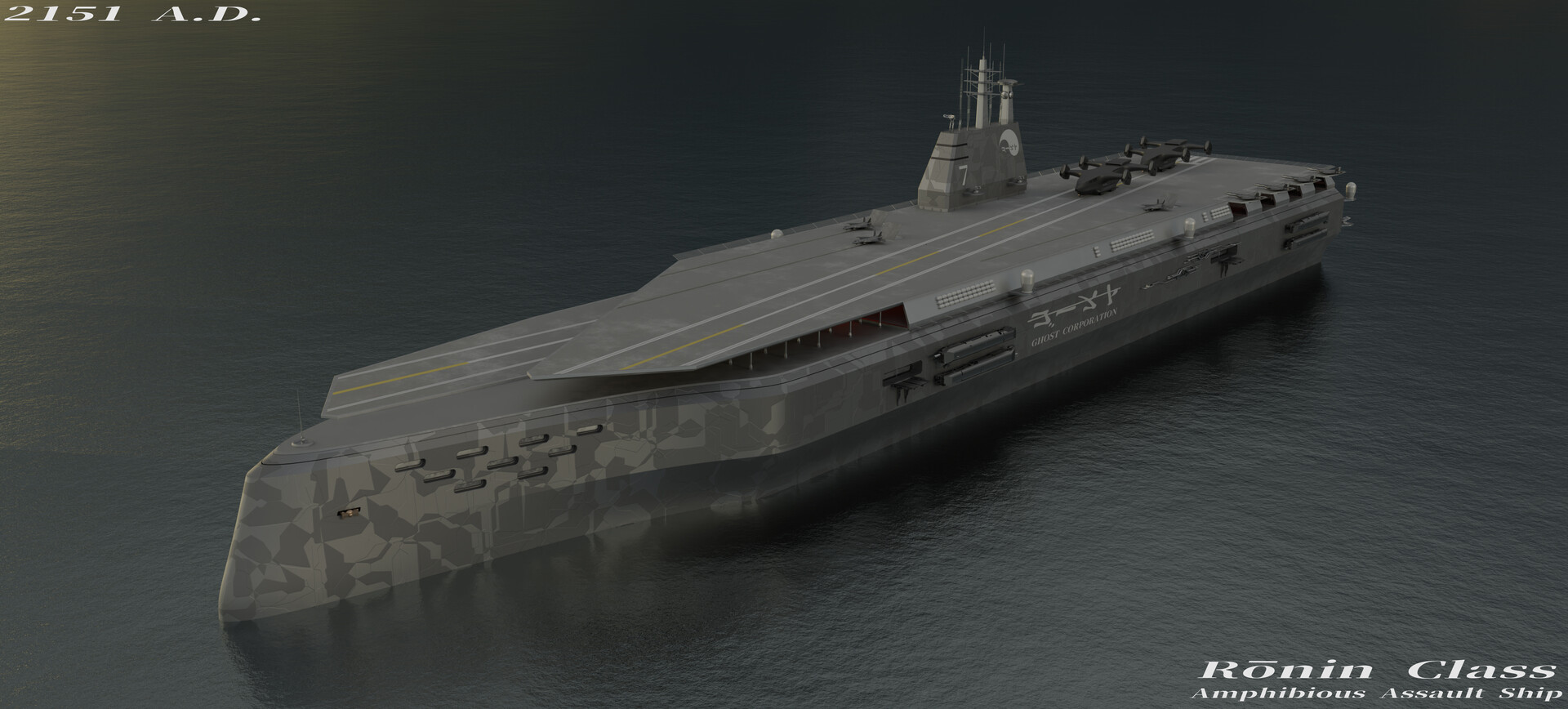The image depicts a computer-generated, futuristic battleship identified as a "Ronin Class Amphibious Assault Ship." The text "2151 AD" is displayed in the upper left corner, indicating the future setting. The ship itself is long and features a flight deck on the top, with at least two visible helicopters or planes positioned on it. The vessel's hull is adorned with a camouflage pattern in gray and khaki green shades. Additional text, including Japanese characters, is present on the side of the ship, though it is too small to decipher. The ship floats on dark, still water, which forms the entire backdrop, enhancing the military and high-tech atmosphere of the scene.